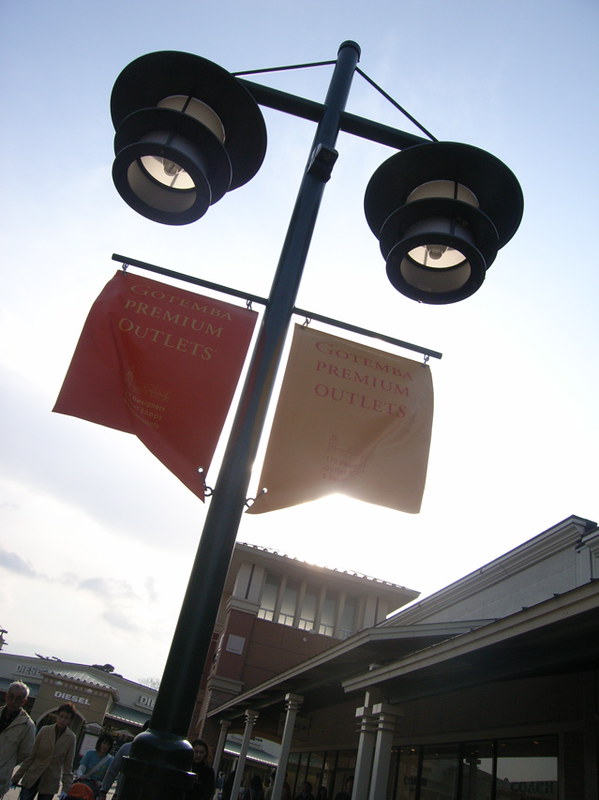The photograph captures an outdoor scene in what appears to be a mall setting, showcasing a streetlamp set against a cloudy yet blue sky that partially reveals the sun. Centrally positioned in the image, the black metal pole of the lamppost branches into a T-shape, supporting two black light fixtures at the top. Hanging from the pole are two banners; the left banner is red with gold lettering that reads "Gotemba Premium Outlets," while the right banner is yellow with red letters bearing the same message. Below the lamppost, a few people, including two men and a woman, are walking. Prominently visible in the background is a building with a storefront sign that reads "Diesel." Another large building featuring a central tower with reflective windows and an adjacent patio is seen to the center right of the image. The atmosphere suggests it could be mid to late evening, given the sun's position and the reflective quality of the windows.